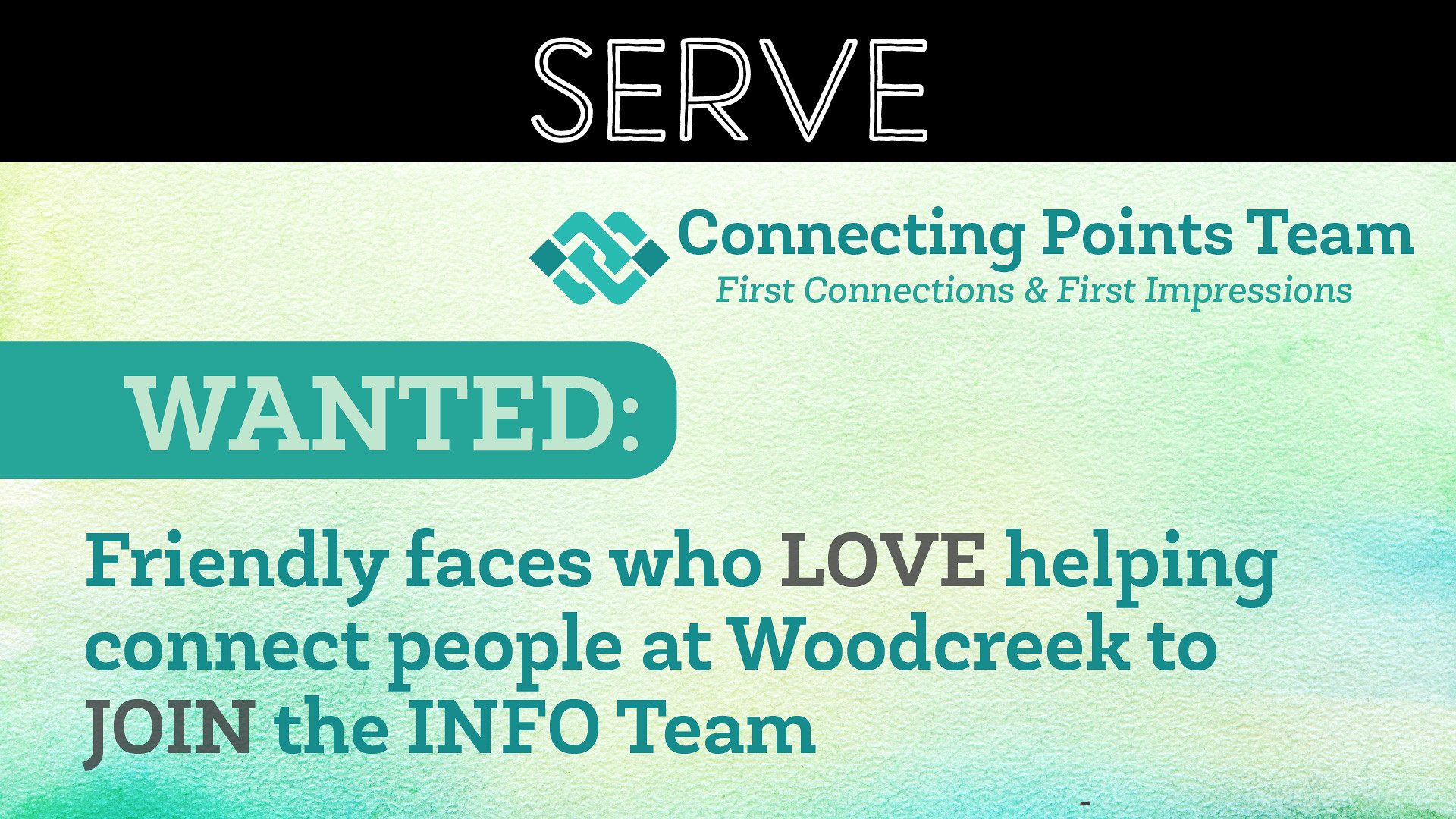The image features an advertisement with a clear emphasis on recruiting friendly individuals for a team. At the very top is a black banner with white text showing the word "Serve." Below this, the background transitions to a greenish-yellow tint. The advertisement text begins with "Connecting Points Team: First Connections and First Impressions" in a lighter green font. Prominently displayed in a large green font, the word "Wanted" stands out, followed by the phrase "Friendly faces who love helping connect people at Woodcreek to join the Info Team." The layout of the text is scattered somewhat unevenly throughout the image, which contains no actual objects—just text and design. The overall theme is light green with touches of white and gray, creating a welcoming and fresh feel typical of recruitment materials.